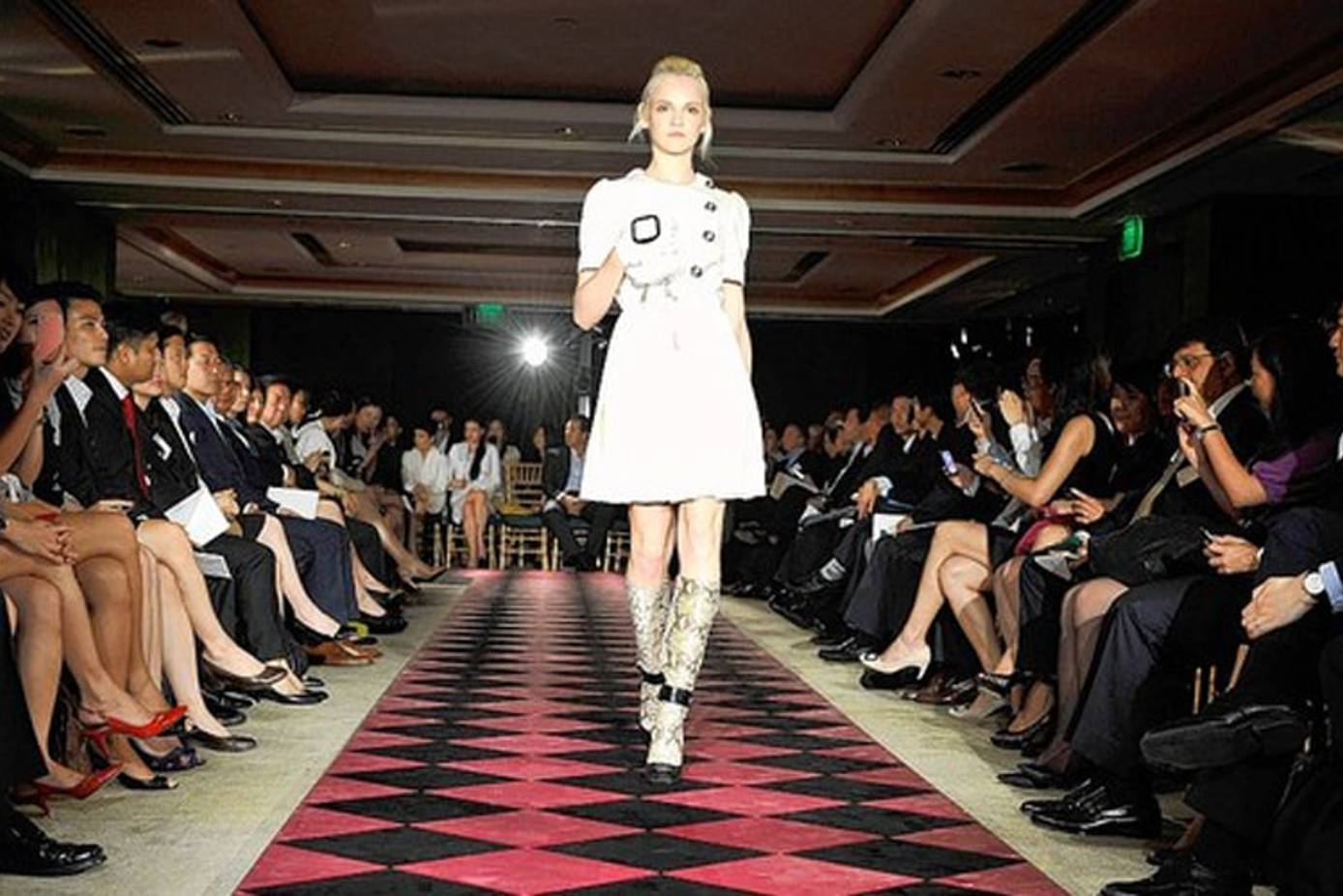In this realistic photograph, a professional model strides down a fashion catwalk in a large, somewhat dim room with approximately 15-foot-high ceilings. The catwalk, which runs through the center of the room, features a distinctive black and red checkerboard pattern created by 12-inch by 12-inch tiles arranged at an angle, contrasting with the concrete-colored floor where the audience is seated. The audience, predominantly Asian, is dressed in formal business attire, mainly black, and flanks both sides of the runway, with additional viewers seated at the back. The model, a slender white woman in her teens or twenties, with blonde hair, advances towards the camera. She is adorned in a vintage-style white dress adorned with black decorations and buttons down the left shoulder, and she may be wearing gloves, holding an object in her right hand that has a black square detail. She completes her ensemble with tall, possibly snakeskin-patterned boots featuring a strap around the ankle and a black sole. Backlighting highlights the scene, ensuring the model stands out amidst the subdued lighting.